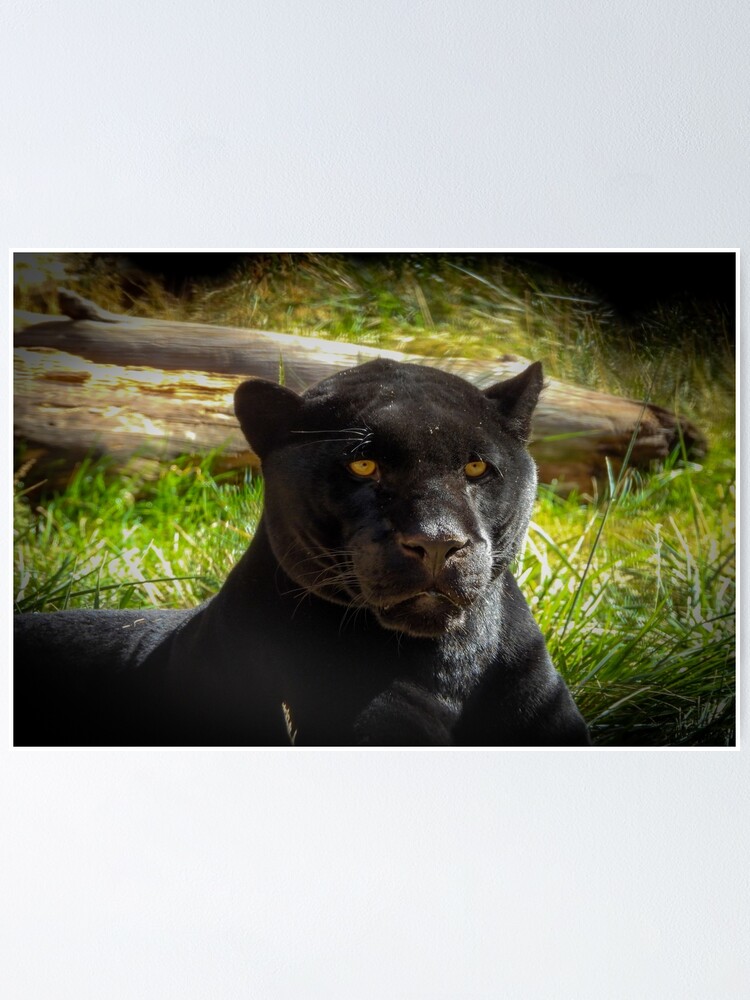This image captures a close-up of a sleek black panther with striking orange eyes, situated slightly off-center and gazing partially toward the camera. The panther's glossy black fur shimmers under a light, creating a faint, illuminated effect that highlights its prominent whiskers. The cat's ears stand erect, and its nose is a lighter shade of black. In the foreground, tufts of green grass and weeds surround the panther, which appears to be lying down, with its chest facing right and its back to the left.

Behind the panther, a partially broken, brown wooden log stretches almost across the entire image, from left to right, with the sun casting lighter and darker shades on its surface. The background features more grass, which appears sharper near the panther but becomes blurrier and wavy towards the back, contributing to an artificial or edited atmosphere. The entire photograph is bordered by a subtle white frame, with a vignette effect darkening the edges, drawing attention to the majestic panther at the center, against what could either be a natural grassy setting or an artificially created backdrop.